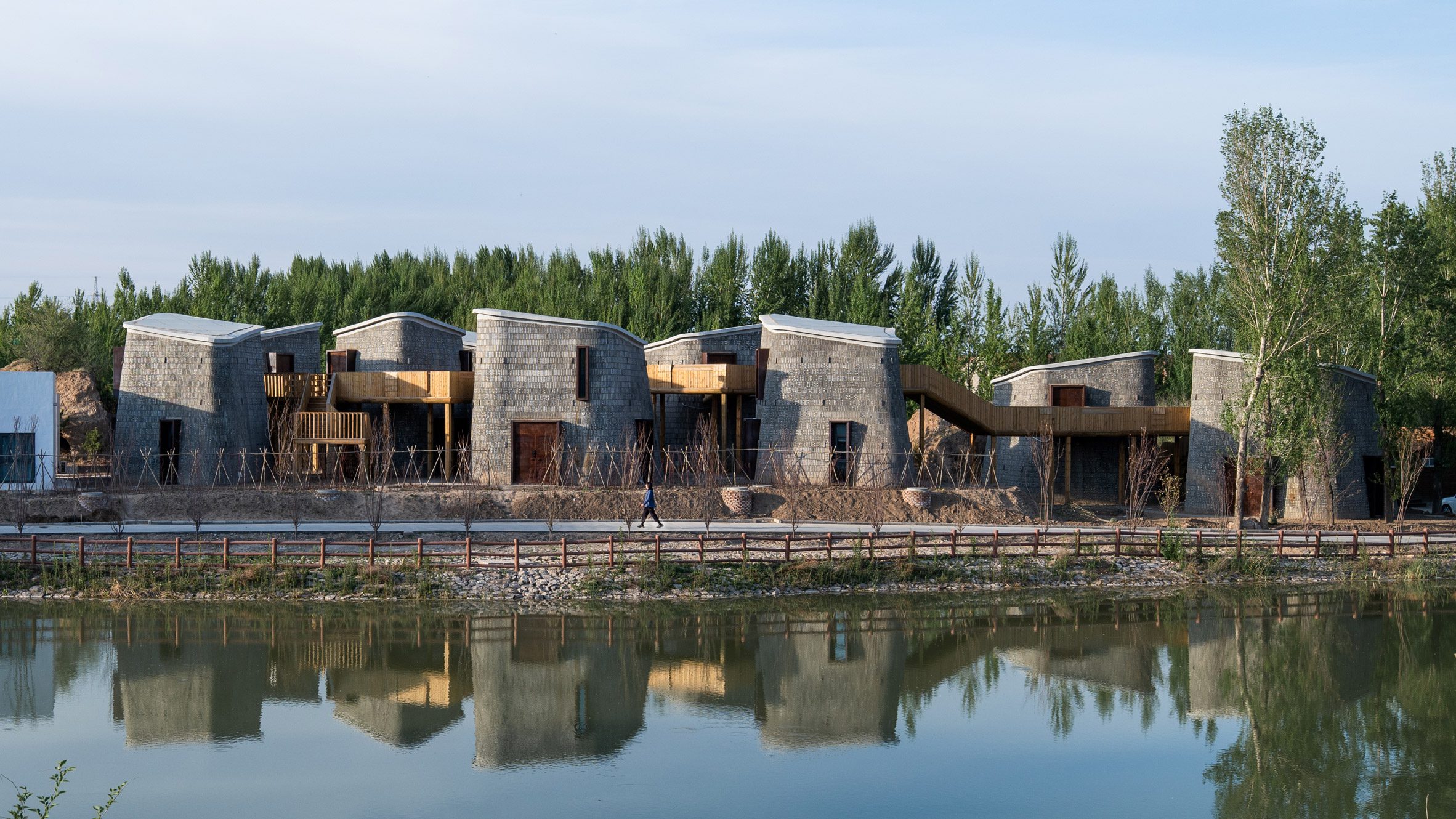The photograph captures a serene waterfront scene featuring a complex of uniquely shaped buildings reflecting on the calm, greenish water. The buildings, constructed from concrete and wood, have an intriguing design with slanted roofs and slightly tilted walls, deviating from traditional cube structures. There are about seven of these interconnected buildings, linked by wooden walkways and stairs. The entire complex is positioned centrally in the image and is bordered by a wooden fence along the rocky, grass-edged shore. A person, dressed in blue and black, is seen walking along a sidewalk in the foreground, adding scale and a sense of life to the scene. The background is lush with green trees under a gray sky, enhancing the tranquil and somewhat mysterious atmosphere of the setting.